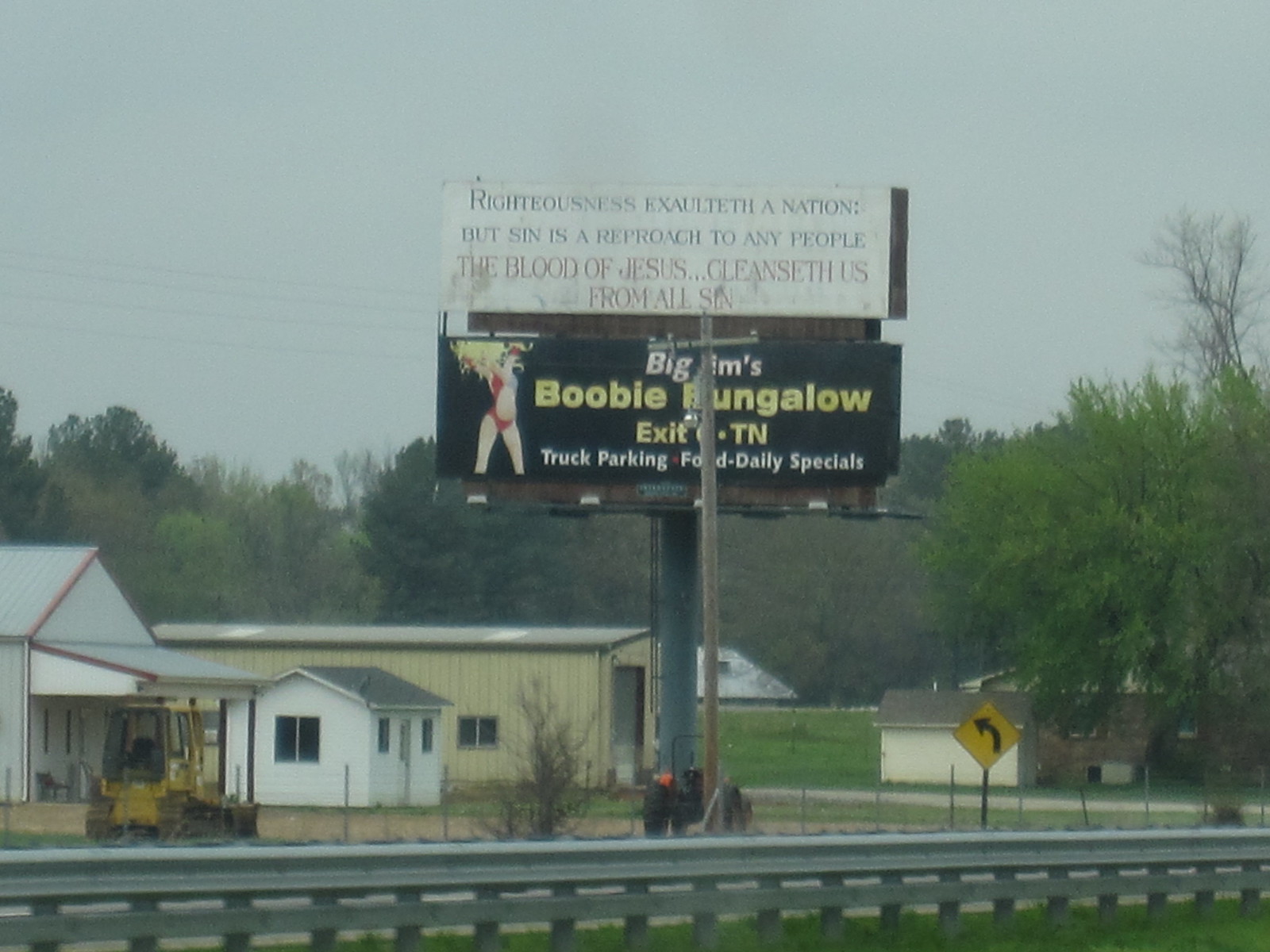The photograph features a rural setting with a prominent metallic pole in the center supporting two contrasting billboards. The top billboard, set against a dirty white background, bears the religious message, "Righteousness Exalteth a Nation, but Sin is a Reproach to Any People. The Blood of Jesus Cleanseth Us from All Sin," in red and blue text. Below it, a black-background billboard advertises "Big Jim's Booby Bungalow, Exit 6, TN" with provisions for truck parking, food, and daily specials. This advertisement includes white and yellow text and a graphic of a blonde woman in a red bikini.

Surrounding the billboards are elements of a rural landscape, including a yellow tractor to the left, a white farmhouse, a smaller white shed, and a larger green shed with a gray roof. In the background, there are numerous green trees and additional white buildings. A road sign indicating a left turn is visible, along with an excavator. The scene is framed by a gray railing at the bottom, suggesting the image is taken from the side of a highway or interstate.